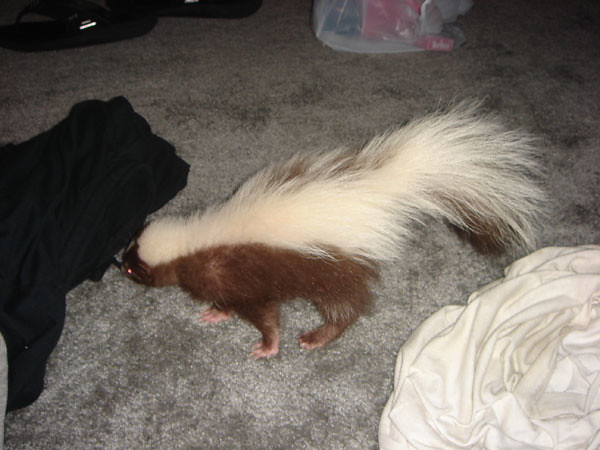The photograph captures a domestic scene featuring a skunk in the middle of a room, appearing to sniff or move towards a crumpled black cloth object on the left side of the picture. The skunk's body showcases contrasting colors: a primarily black back, a brown lower half, and light tan feet, with its fluffy tail extending with a prominent white streak running from its head to its tail end. The setting is in a home, evidenced by the grayish-black carpet covering the floor, which transitions to darker gray when rubbed. In the bottom right corner, a bunch of white sheets is folded neatly, while the background reveals a white, slightly see-through bag containing items in blue and pink. The skunk is central to the image, visibly showing three of its four paws, adding to the detailed depiction of this curious encounter within a cozy indoor environment.